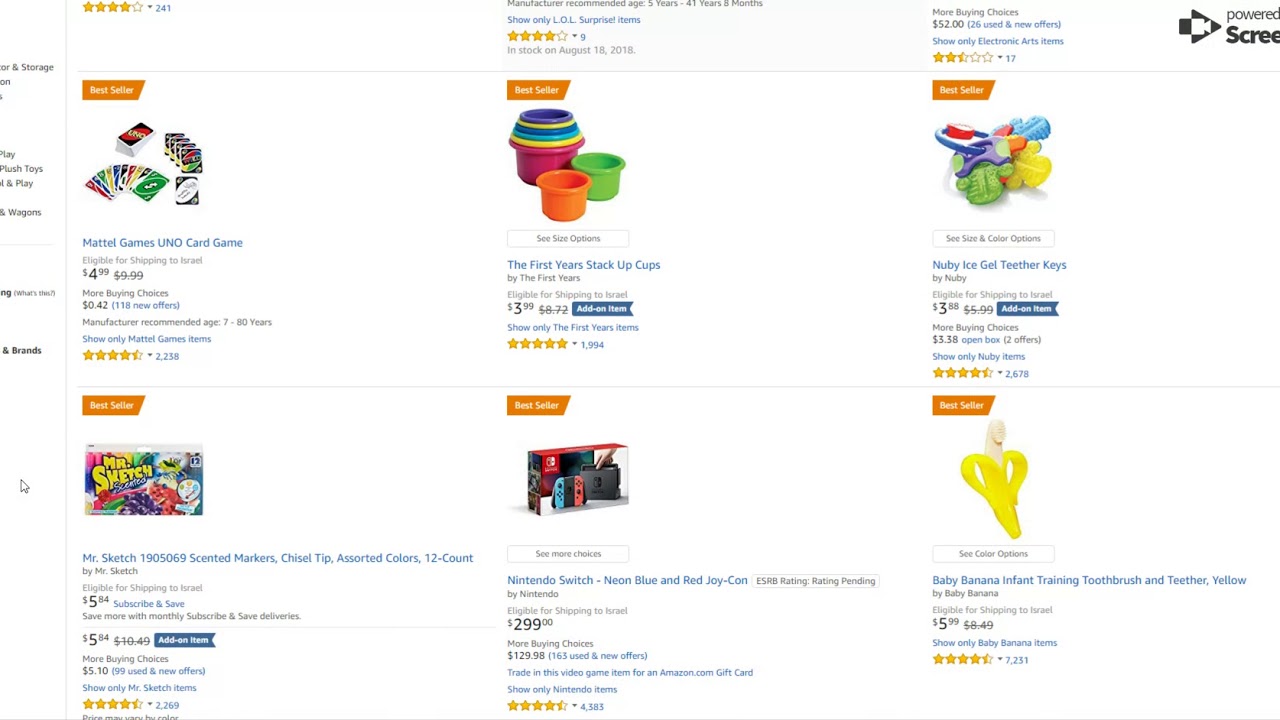This image appears to be a screenshot from an online shopping page, potentially Amazon, although the exact platform is not confirmed. The visible portion showcases six products arranged in two rows of three, with more items extending above beyond the visible area.

1. **First Product (Top Left)**
   - **Title**: Best Seller - Mattel Games Uno Card Game
   - **Details**: 
     - Price: $4.99 (previously $9.99)
     - Additional Offers: More buying choices starting at $0.42, with 118 new offers
     - Age Recommendation: Manufacturer recommended age 70 to 80 years
     - Shipping: Eligible for shipping to Israel
     - Ratings: 4.5 stars from 238 reviews
     - Additional Info: Option to filter by "Show only Mattel Games items" highlighted in blue

2. **Second Product (Top Center)**
   - **Title**: Best Seller - The First Years Stack-Up Cups by The First Years
   - **Details**: 
     - Price: $3.99 (previously $8.72)
     - Add-On Item: Yes
     - Shipping: Eligible for shipping to Israel
     - Ratings: 5 stars from 1,994 reviews
     - Additional Info: Option to filter by "Show only The First Years items" highlighted in blue

3. **Third Product (Top Right)**
   - **Title**: Best Seller - Nuby Ice Gel Teether Keys by Nuby
   - **Details**: 
     - Price: $3.88 (previously $5.99)
     - Additional Offers: More buying choices starting at $3.88, with open box options listed
     - Add-On Item: Yes
     - Shipping: Eligible for shipping to Israel
     - Ratings: 4.5 stars from 678 reviews
     - Additional Info: Option to filter by "Show only Nuby items" highlighted in blue

The page gives a clear indication of the popularity and affordability of these products, emphasizing their ratings, available offers, and shipping eligibility.